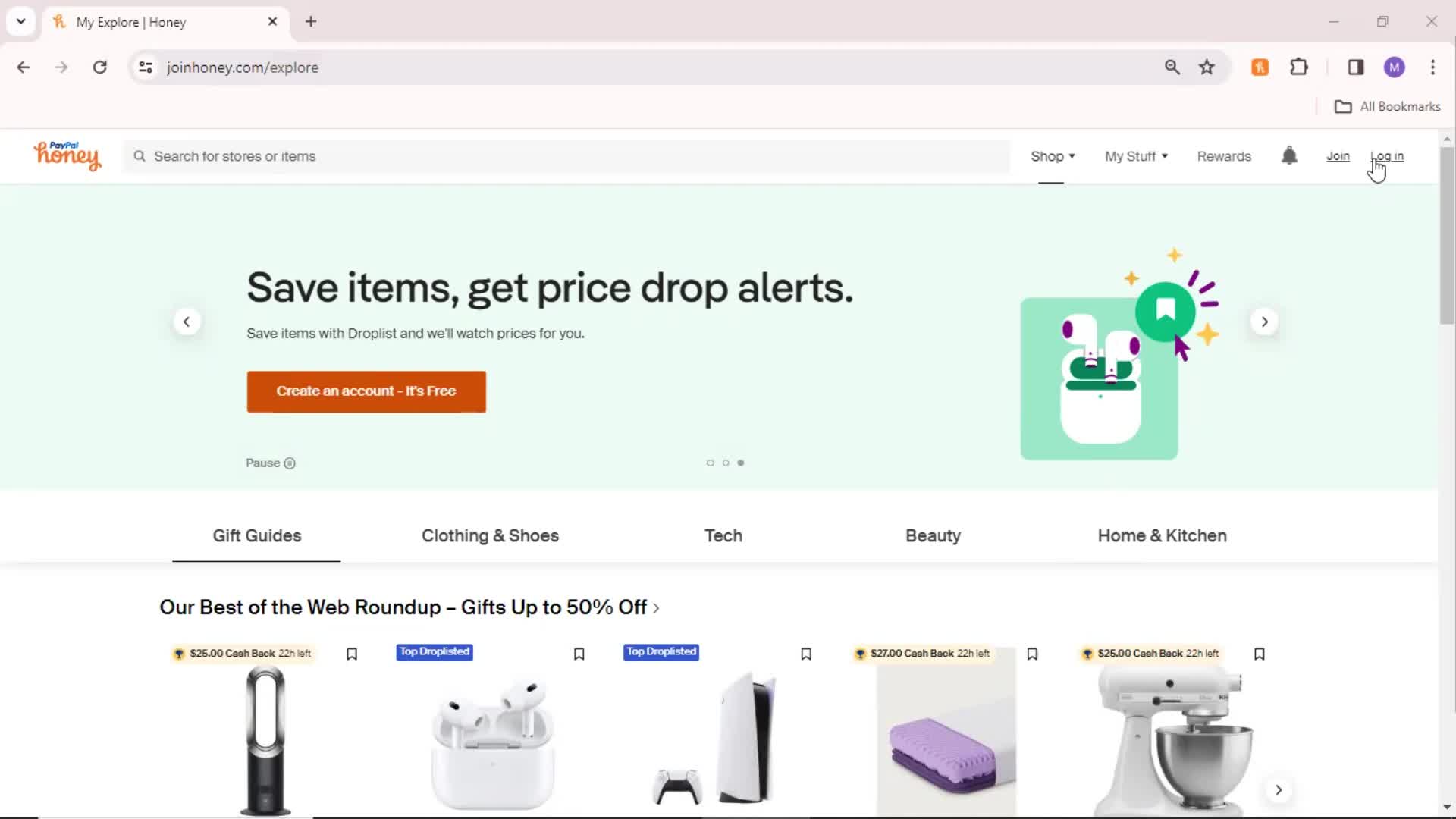The webpage displayed is for MyExploreHoney, accessible via joinhoney.com/explore, and is being viewed on the Google Chrome browser. At the top left corner of the page, there are navigational options: back, forward, and refresh. Below these options, the logo for PayPal is present, indicating an association with Honey, followed by the Honey logo itself. There is a search bar prompting users to "search tours for our items."

The main navigation menu includes the sections: Shop, My Stuff, Rewards, Notifications, Join, and a Login button, with the cursor currently hovering over the Login button, changing it to a hand symbol. A highlighted orange box with white text reads, "Create an account, it's free." Just below, there is information about saving items to get price drop alerts and using the drop list feature to monitor price changes.

On the upper right-hand side of the image, a purple cursor is shown selecting a bookmark option next to a picture of a pair of earbuds. Below this, more menu options are visible, including Gift Guides, Clothing Stores, Tech, Beauty, and Home & Kitchen, arranged horizontally from left to right.

The webpage also features images of various sale items that customers can watch, including earbuds, a PlayStation 5, cashback options for a bed, and a mixer/blender. This page serves as one of the primary interfaces for Honey's discount program, showcasing a variety of items and shopping tools available to users.